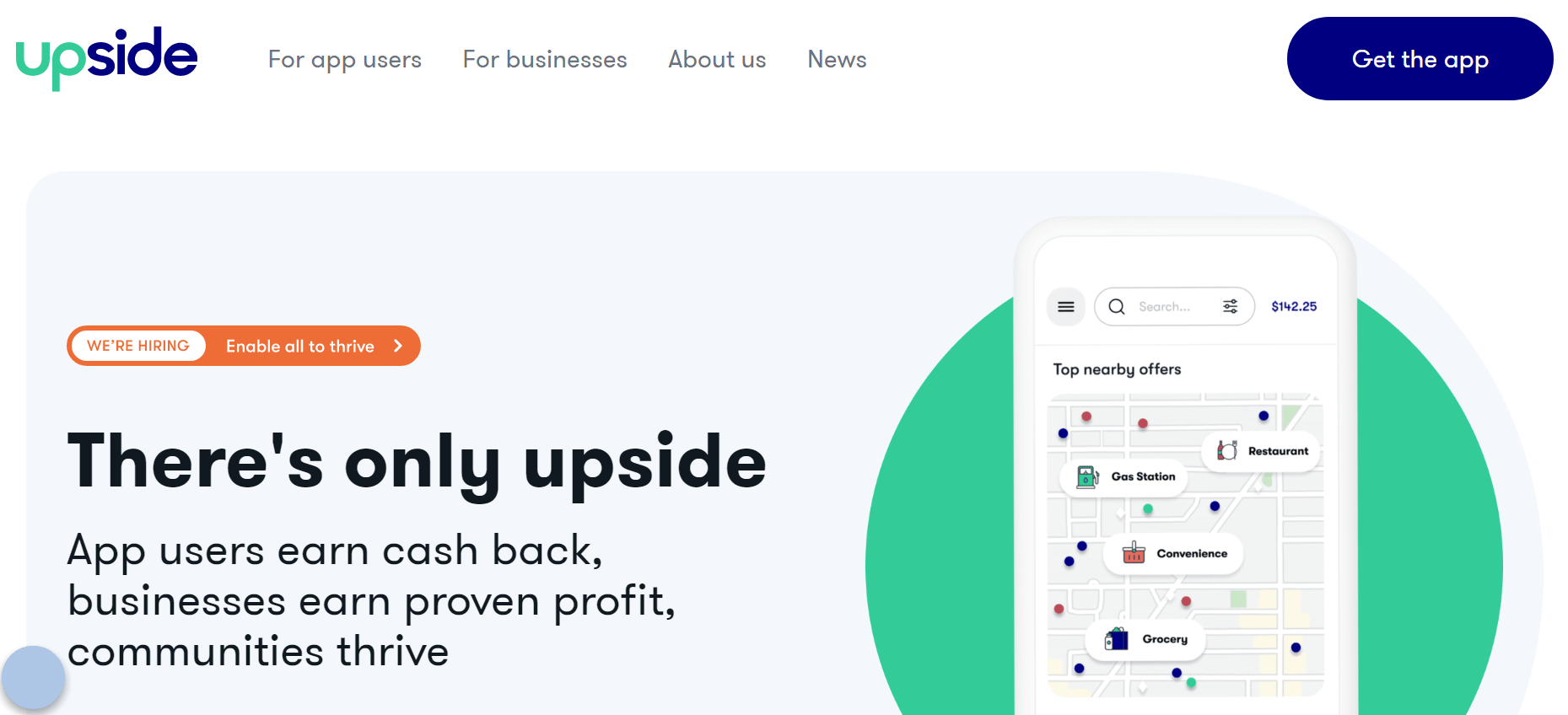Screenshot of the Upside App Homepage: This detailed screenshot captures the main webpage of the Upside app, designed for users to save money on gas, earn cash back, and receive rewards at various stores and restaurants. The top left corner prominently features the Upside logo and name, with a navigation menu including options for 'App Users,' 'Businesses,' 'About Us,' and 'News.' On the upper right corner, a blue 'Get the App' button directs users to download the app from the appropriate app store. Below the navigation bar is a prominent graphic on a bluish background with a green circle. In front of this circle is an illustration of a smartphone displaying a map covered in location pins, symbolizing various places where savings can be achieved. To the left of this visual, bold text reads, "There's only Upside." Accompanying this statement, smaller subtext informs users that "App users earn cash back, businesses earn proven profit, and communities thrive." This clean and organized interface reflects the essential features and value propositions of the Upside app.